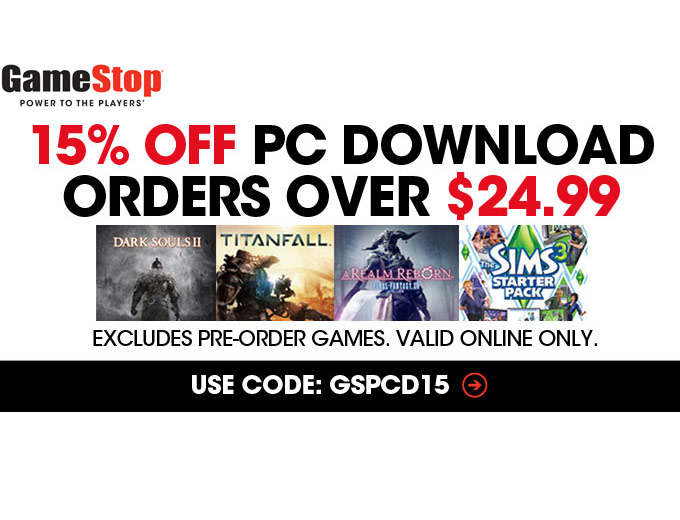This is a detailed screenshot of a GameStop advertisement. In the upper left corner, the GameStop logo is prominently displayed with the slogan "Power to the Players" directly beneath it. Below the slogan, a bold red text announces "15% OFF" and in black text it specifies "PC download orders over $24.99," with the price "$24.99" in red for emphasis. 

The advertisement showcases four featured games: Dark Souls 2, Titanfall, Final Fantasy XIV: A Realm Reborn, and The Sims 3 Starter Pack. Additionally, it notes "Excludes pre-ordered games" and "Valid online only," with the promotional code "GCPCD15" highlighted for customers to use. A red arrow points to the right toward this code, emphasizing its importance. Along the bottom of the advertisement, there is a black bar which further highlights the text mentioning The Sims 3 Starter Pack.